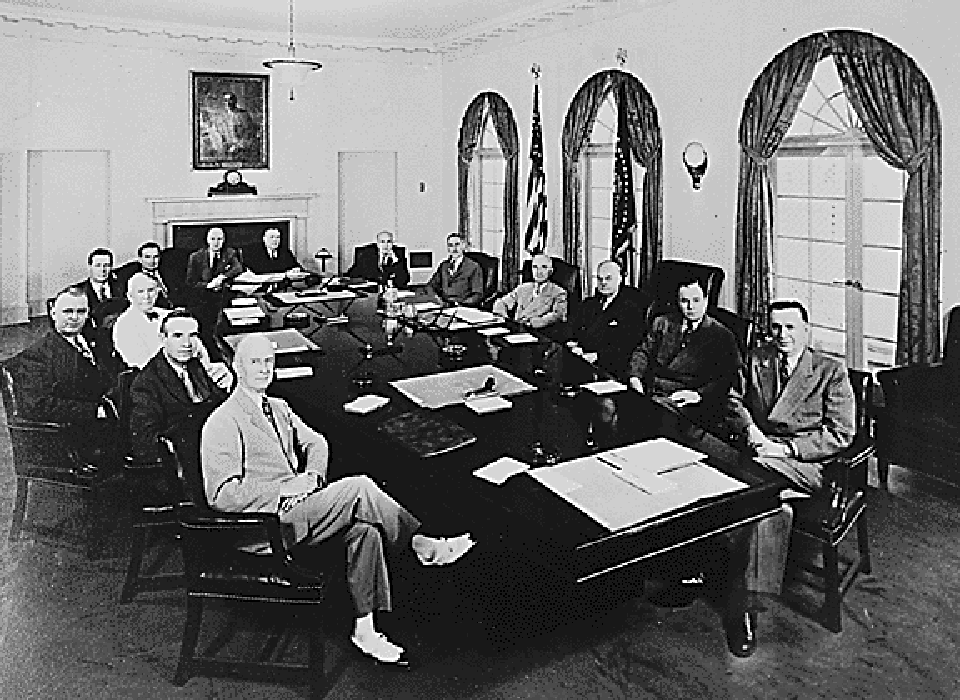The vintage black and white photograph depicts a distinguished gathering of men, all dressed in suits and ties, seated around a large conference table in the White House’s Breathing Room. Central to the image, and towards the right, is President Harry S. Truman, recognizable in a lighter colored suit. There are approximately fourteen men in total, arranged along both sides of the table, some sitting in front of arched windows with dark drapes, and others positioned on the opposite side. The table in front of them is strewn with papers and notebooks, and in front of the President is a pen set. The room features upholstered wooden chairs and elegant furnishings, including a central fireplace with a painting and a clock on the mantel. The photograph, taken from an elevated angle, captures the men all looking directly at the camera, suggesting a formal, posed setting. The lighting implies it was taken during the daytime, further enhancing the image's historic and somewhat solemn atmosphere.